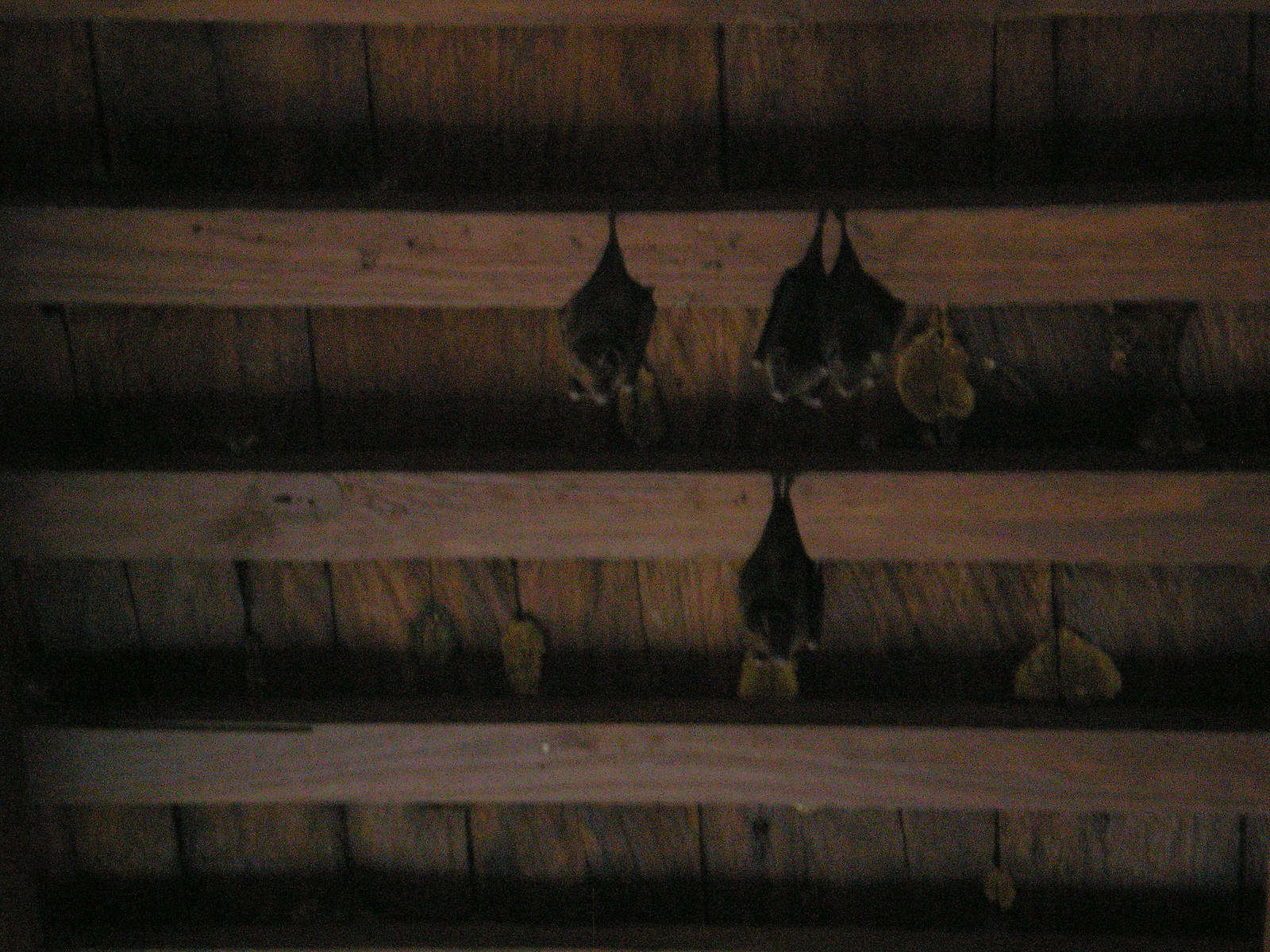The photograph depicts the dimly lit interior of a timber-wood cabin roof, featuring multiple wooden beams spanning horizontally and vertically. The focus is on four bats hanging upside down from the thick wooden rafters. Three bats are clustered together on the uppermost horizontal beam, while a solitary bat dangles from a middle beam. The cabin's overall darkness, possibly lit only by a dim candle, accentuates the mold's yellow and dark brown hues on the aged wood. The bats, appearing brown or black in the shadowy light, seem restful and undisturbed in their eerie, secluded roost.